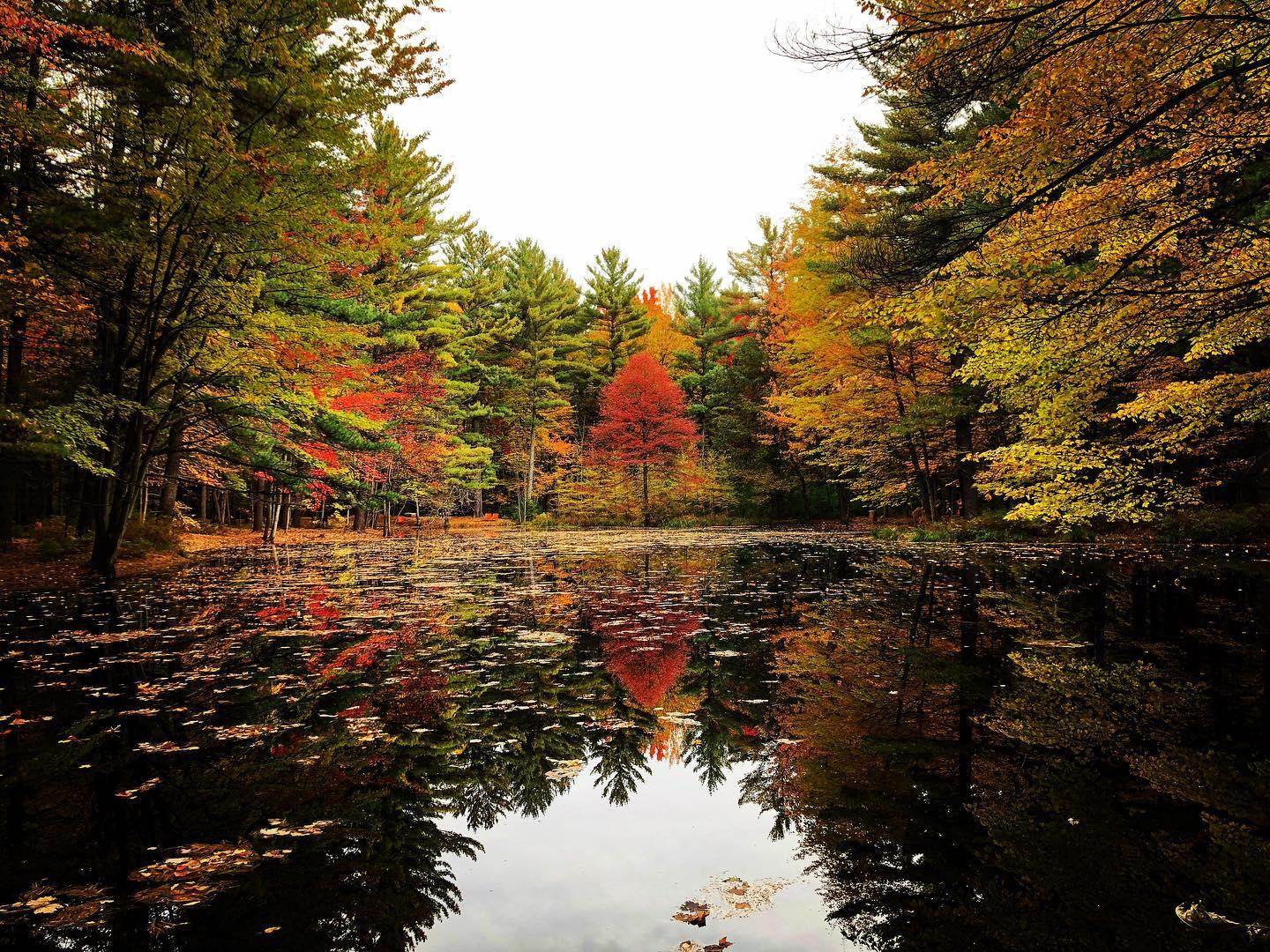This stunning nature scene captures a serene autumn landscape centered around a tranquil lake or pond. The water is so still it resembles glass, perfectly reflecting the surrounding trees and a sliver of sky that peeks through the canopy at the top of the image. The season is unmistakably fall, with an array of foliage in vibrant hues of red, orange, yellow, green, and even some pinks. Dominating the center is a striking small tree ablaze in fiery red, drawing the eye with its dramatic color that contrasts with the varied shades of the other trees. Surrounding the water on all visible sides are trees of various heights, including pines and deciduous trees, some still clinging to green leaves while others showcase yellows, golds, and oranges. The surface of the water is speckled with fallen leaves, adding texture and a slightly murky appearance. Overall, the reflection of the colorful foliage in the calm, leaf-strewn water creates a mesmerizing and harmonious autumnal tableau.